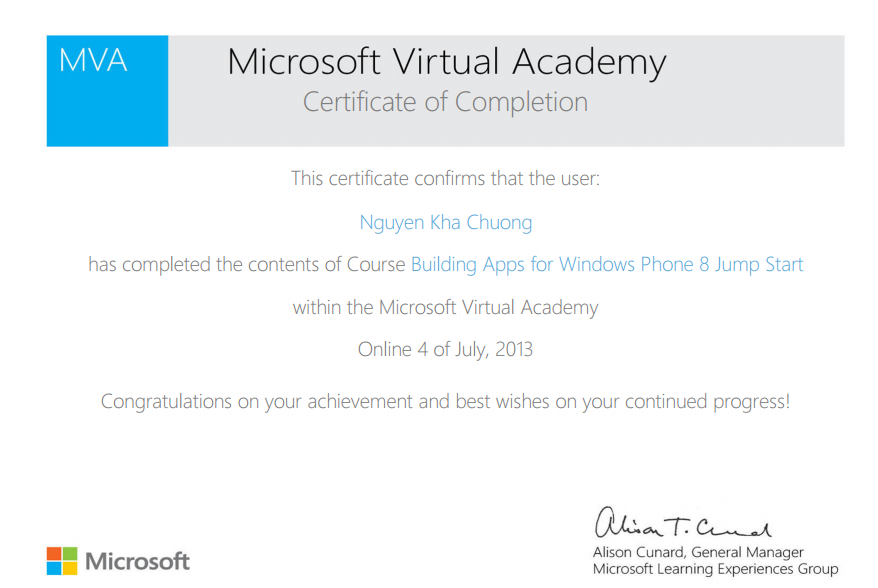The image depicts a certificate from Microsoft Virtual Academy, prominently featuring the text "Microsoft Virtual Academy" at the top. The title "Certificate of Completion" is displayed in gray text on a pale gray background in the center. In the upper left corner, the acronym "MVA" is shown in white text against a blue box.

The certificate confirms that the user, Nagim Ka Chong, has successfully completed the "Building Apps for Windows Phone 8 Jumpstart" course. The completion date is specified as July 4th, 2013. It extends congratulations on the user's achievement and best wishes for continued progress. The certificate is signed by Alison Kinnard, General Manager of the Microsoft Learning Experiences Group. 

Additionally, the bottom left-hand corner of the certificate displays the Microsoft logo, consisting of four colored squares (red, light green, yellow, and blue, arranged clockwise), followed by the word "Microsoft."